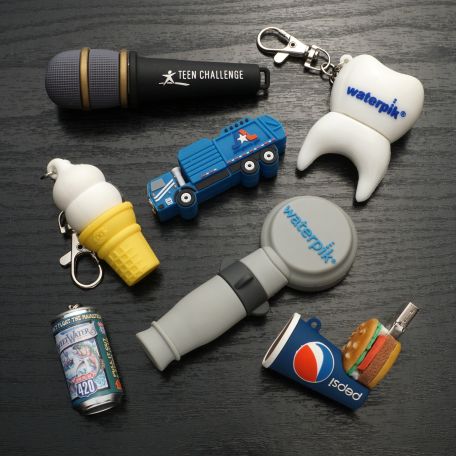The image displays a variety of seven keychains and trinkets spread across a dark brown, wood-grain desktop. In the upper left corner, there is a mini microphone with the body labeled "Teen Challenge" in white, distinguished by its black base, two gold bands, and a silver microphone piece. Adjacent to the right is a keychain shaped like a giant tooth, branded "Waterpik" in blue. Below the tooth keychain is another gray microphone keychain also marked "Waterpik." Toward the center, a keychain takes the form of a small, blue toy trash truck. Next to it on the left, there is a keychain modeled as a vanilla ice cream cone with a yellow base, reminiscent of a Dairy Queen treat. Below these, a keychain shaped like a blue Pepsi cup with an attached cheeseburger sits to the bottom right. Additionally, there is a fallen keychain featuring a mini beer can, and another resembling a bottle of water labeled "420."